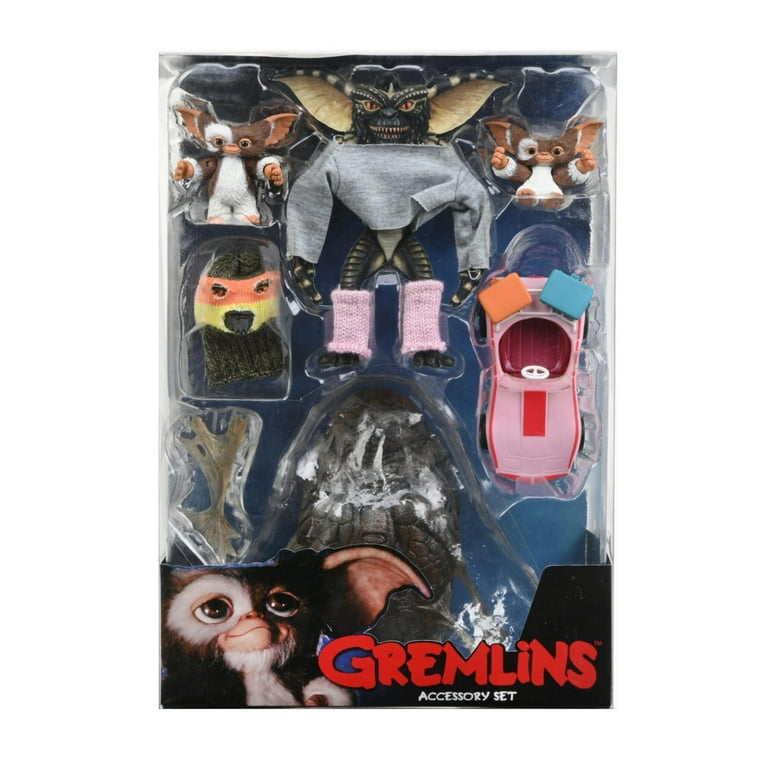The image depicts a "Gremlins Accessory Set" toy product still in its box. The packaging is a sealed, molded plastic that is difficult to open. Prominently displayed at the bottom is the text "Gremlins" in large red letters, with "accessory set" in smaller white text. The packaging illustration features a fur-covered creature with large eyes, long ears, and a bald nose and mouth area, similar to the character Gizmo from the movie, sporting patches of brown and white fur. The enclosed accessories include miniature versions of various gremlins, notably a large black gremlin wearing pink leg warmers and a gray sweatshirt. Additional items include a ski mask, a pink toy car with suitcases hanging off the back, and other miscellaneous accessories, all set against a plain white background.